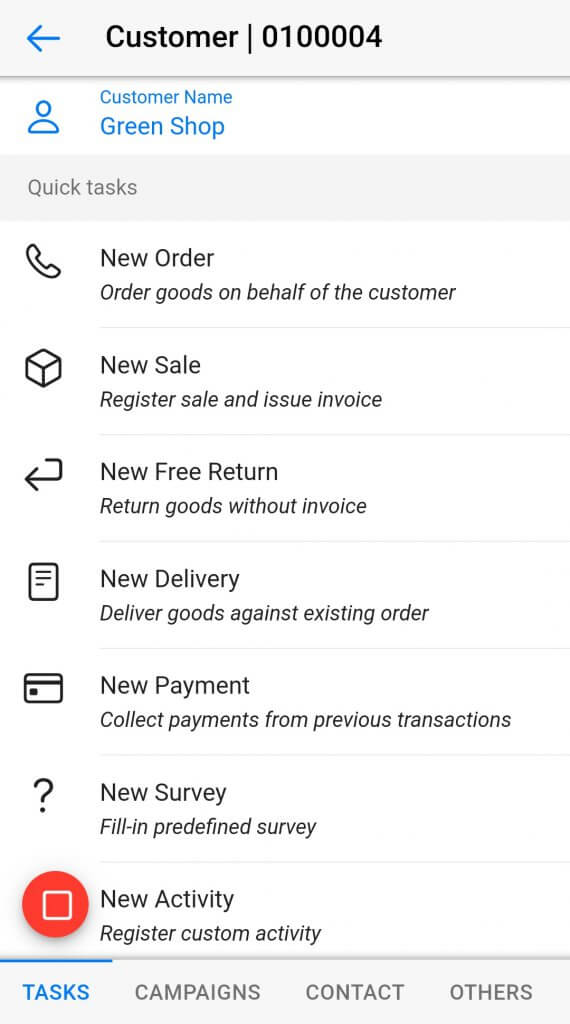This image showcases a screenshot from a customer interface. In the upper left corner, there is a back arrow button, situated to the left of the "Customer" label. Below the label, a unique customer identification number "01000004" is displayed. Directly beneath this, there is a "Customer Name" field, which is set to "Green Shop." Adjacent to the "Customer Name" field on the left side, there is a default profile silhouette icon, all elements are highlighted in blue.

Below the blue section is a gray bar containing the phrase "Quick Test" in gray font. Underneath this bar, there is a vertical list of seven items, each labeled as follows:
1. New Order,
2. New Sale,
3. New Free Return,
4. New Delivery,
5. New Payment,
6. New Survey,
7. New Activity.

These items are stacked one above the other, representing various actions available to the customer.